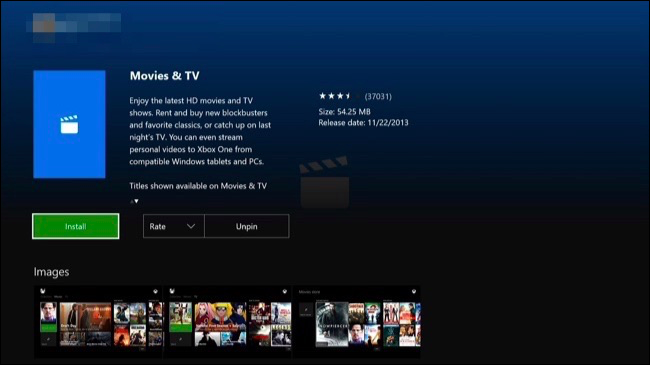The image features a computer app with a sleek dark blue background that seamlessly fades into black. The top of the interface prominently displays the title “Movies and TV,” inviting users to enjoy the latest HD movies and TV shows. The app offers options to rent or buy new blockbusters and favorite classics, as well as catch up on last night's TV episodes. A unique feature allows users to stream personal videos to an Xbox One from compatible Windows tablets and PCs.

The title, "Movies and TV," is showcased on a lighter blue background, accompanied by a white director’s cut icon. To the right of this title, the app has received an average rating of three and a half stars based on 37,031 reviews. Additional information indicates that the app's file size is 54.25 megabytes, and it was released on November 22, 2013. Users have options to install, rate, or unpin the app.

Below these details, the interface displays images of various movies and TV shows, organized into different categories. The first category features a solo male figure, possibly Leonardo DiCaprio, although the image is slightly unclear. The second category contains multiple people. Another category includes a cartoon or anime. Lastly, there appears to be a group that combines thrillers and comedies, suggesting that the movies and TV shows are sorted based on thematic elements.

Overall, the detailed layout and functionality of the app create an engaging experience for users looking to explore a variety of film and TV content.